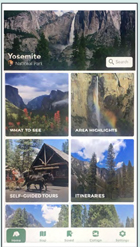The image appears to be a screenshot from a cell phone, displaying information related to Yosemite National Park. The layout is in portrait orientation, clearly divided into several rows.

**Top Row:**
- Dominated by a single rectangular section stretching across the width of the screen.
- The background showcases a majestic scene featuring light gray rocks, a waterfall, and a body of water.
- In the lower left corner of this image, the word "Yosemite" is written in white text.
- Directly below it, an orange icon appears with the words "National Park" in white.
- To the right, a rectangular search field displays a gray magnifying glass icon and the placeholder text "Search."

**Second Row:**
- Composed of two side-by-side square panes.
- **Left Pane:** 
  - Background features a vibrant blue sky with clouds, mountainous terrain, and foreground vegetation including red flowers.
  - At the bottom, white text reads "What to See."
- **Right Pane:**
  - Background presents beige rocks and cliffs, with a waterfall coursing down the center, accompanied by a rainbow.
  - The text at the bottom, in white, reads "*indistinguishable first word* Highlights."

**Third Row:**
- Also consists of two adjacent square panes.
- **Left Pane:**
  - Features a picturesque background with a two-story house with a pitched roof, trees, and a blue sky.
  - In the foreground, a buggy pulled by black horses moves toward the right.
  - The bottom text identifies it as "Self-Guided Tours" in white.
- **Right Pane:**
  - Showcases an impressive landscape of blue sky, white clouds, cliffs, mountains, and two tall pine trees.
  - Labeled "Itineraries" at the bottom in white text.

**Fourth Row:**
- Only partially visible, featuring two side-by-side panes.
- Both panes highlight outdoor scenes with blue skies and trees.
- The very bottom of the screen shows a light-colored band with several green icons on a white background. The icons and the text beneath them are unreadable.

This detailed view provides a comprehensive understanding of the presented information and layout in the image.